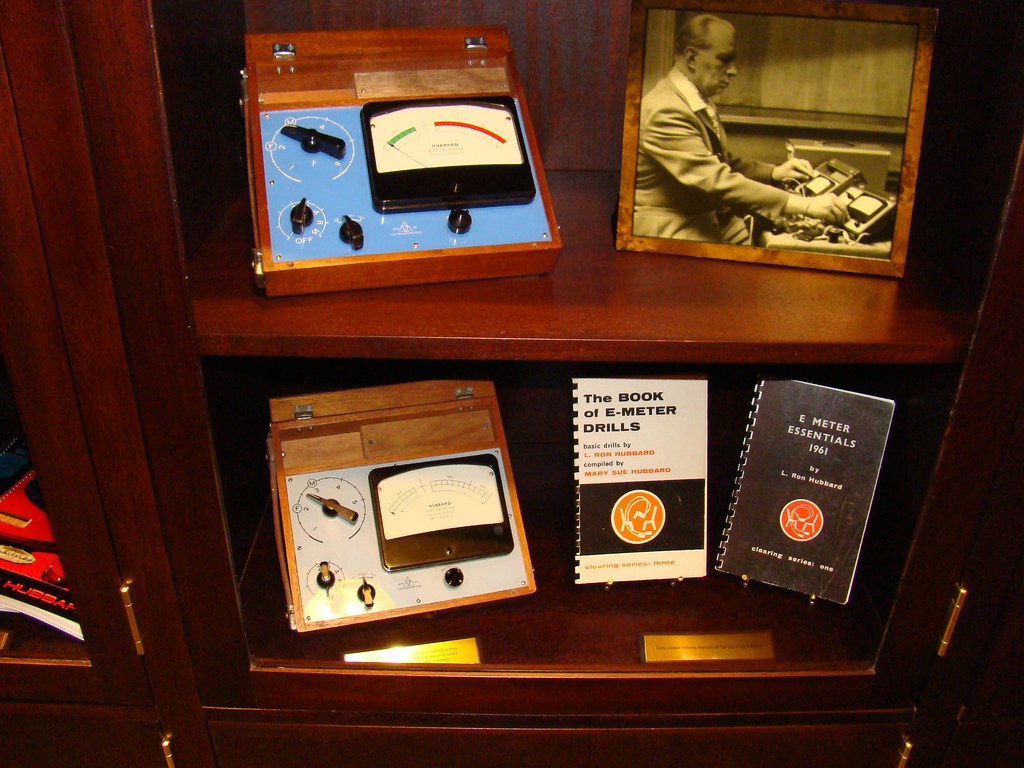This image showcases a wooden display cabinet with two shelves, protected by a glass case, displaying important historical artifacts related to E-Meters. On the top shelf, to the right, there is a vintage black-and-white photograph of a prominent man, likely L. Ron Hubbard. He is seen dressed in a suit jacket and white collared shirt, adjusting dials on two E-Meters with an intense expression, set against a wooden wall backdrop. To the left of the photo is a more modern-looking E-Meter with a wooden base and a blue plate, featuring four black dials with white indicators and a meter that changes from green to yellow to red.

The bottom shelf houses an older E-Meter characterized by a simpler design. This device, also set on a wooden base but with a white plate, has three dials and a meter gauge. Next to it are two books. The first book, which is white, titled "The Book of E-Meter Drills: Basic Drills" by L. Ron Hubbard and compiled by Mary Sue Hubbard, features an orange logo depicting a machine with two chairs and connecting wires with handles. The second book, black in color, is titled "E-Meter Essentials" from 1961.